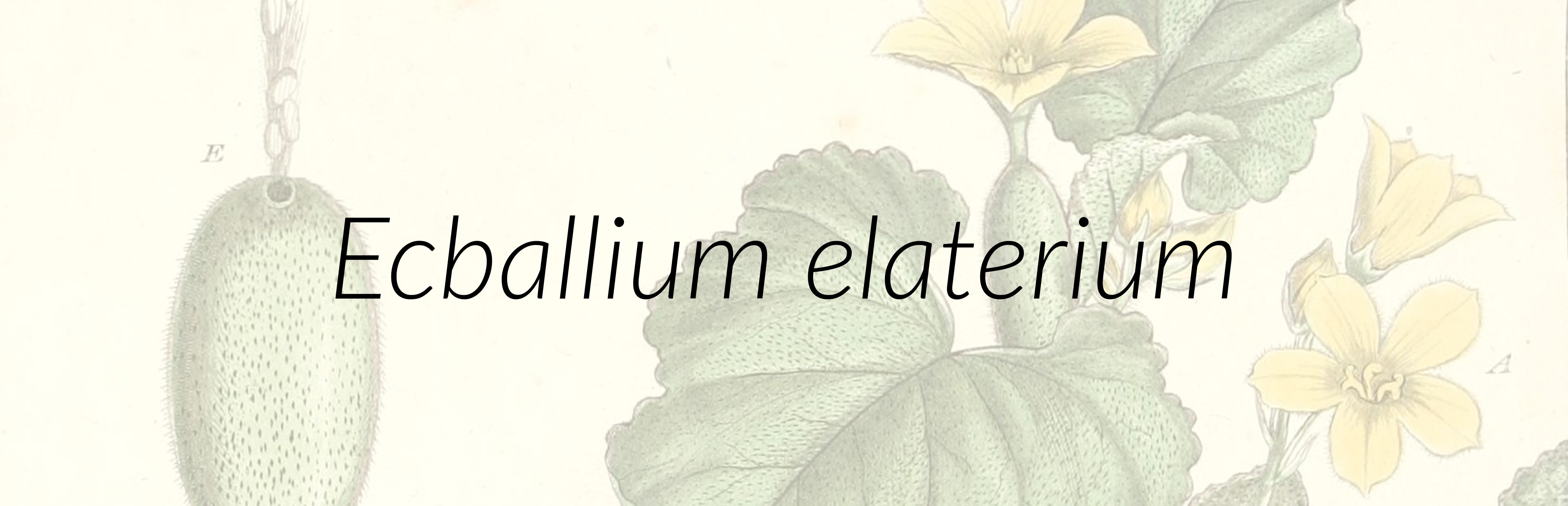The image features a pastel pink background with a slight white overlay, creating a soft, pale appearance. On the left side, there's an intriguing object resembling an oblong, very light green bulb or pod, dotted with a darker hue and having a chain emerging from a small hole at its top. Towards the right side of the image, stands a lush green plant with large, veined leaves. The plant boasts several yellow flowers: two are fully open, one is halfway open, and there are additional buds. The vibrant yellow flowers, slightly darker than the background, each have five distinct petals. Below the flowers, at the base, another light green bulb similar to the one on the left can be seen. The words "Ectbalium elaterium" are written in black, completing the composition of this detailed, vibrant picture that may form part of an advertisement or magazine page.